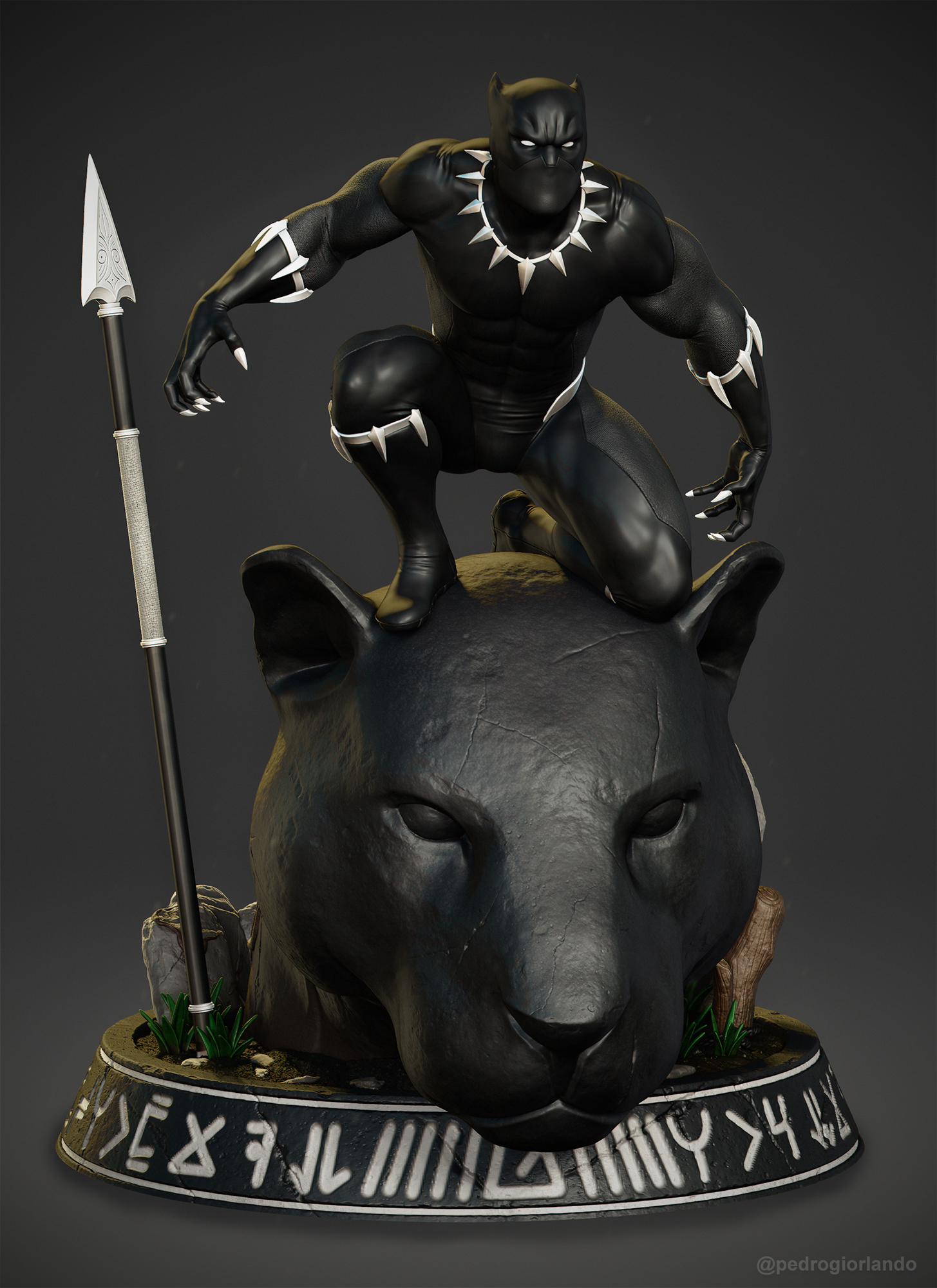The image displays a detailed figurine depicting an imposing black panther motif. At the focal point sits a large, black panther head, centrally positioned and facing the viewer. Perched atop this head is a crouching black panther figure, resembling a black man adorned in a panther-like costume. This figure features fierce white claws, white highlights around the neck, knees, and fingertips, and wears a mask. He also has white fanged armbands and a matching white fanged necklace, adding to his menacing appearance. His left knee is bent resting on the panther's head, while his right foot is firmly planted, and his arms are stretched out as if ready for action. To the left of this primary figure is a spear with distinctive white accents, standing upright. The entire assembly rests on a circular base embellished with grayish rocks, greenery, and hieroglyphic-like symbols, though the text is indecipherable. The predominant colors in the image are black, white, gray, green, and brown, with a gray background accentuating the overall composition.